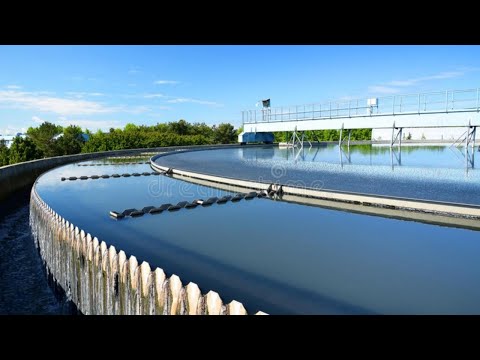The image depicts an outdoor, circular water treatment facility under a clear blue sky punctuated with white clouds. The central feature is a large, round tank filled with dark blue or gray water, bordered by a ring-like structure that encloses smaller sections within it. Long arms, possibly rotating mechanisms, extend from the central part of the tank, suggesting they circulate the water. Above this tank, a white, metal walkway bridges across, allowing for inspection or maintenance, and is supported by guardrails and stands.

The tank itself is enveloped by a white picket fence which adds to the structural division within the water. On the right side, a white industrial building can be seen in the background, while lush green trees frame the left side, creating a natural backdrop to the mechanical setup. The facility's elevated position allows for a perspective that aligns with the tree line, hinting at its height above ground level. This infrastructure combines functionality with a hint of design, making the setting both practical and visually interesting.